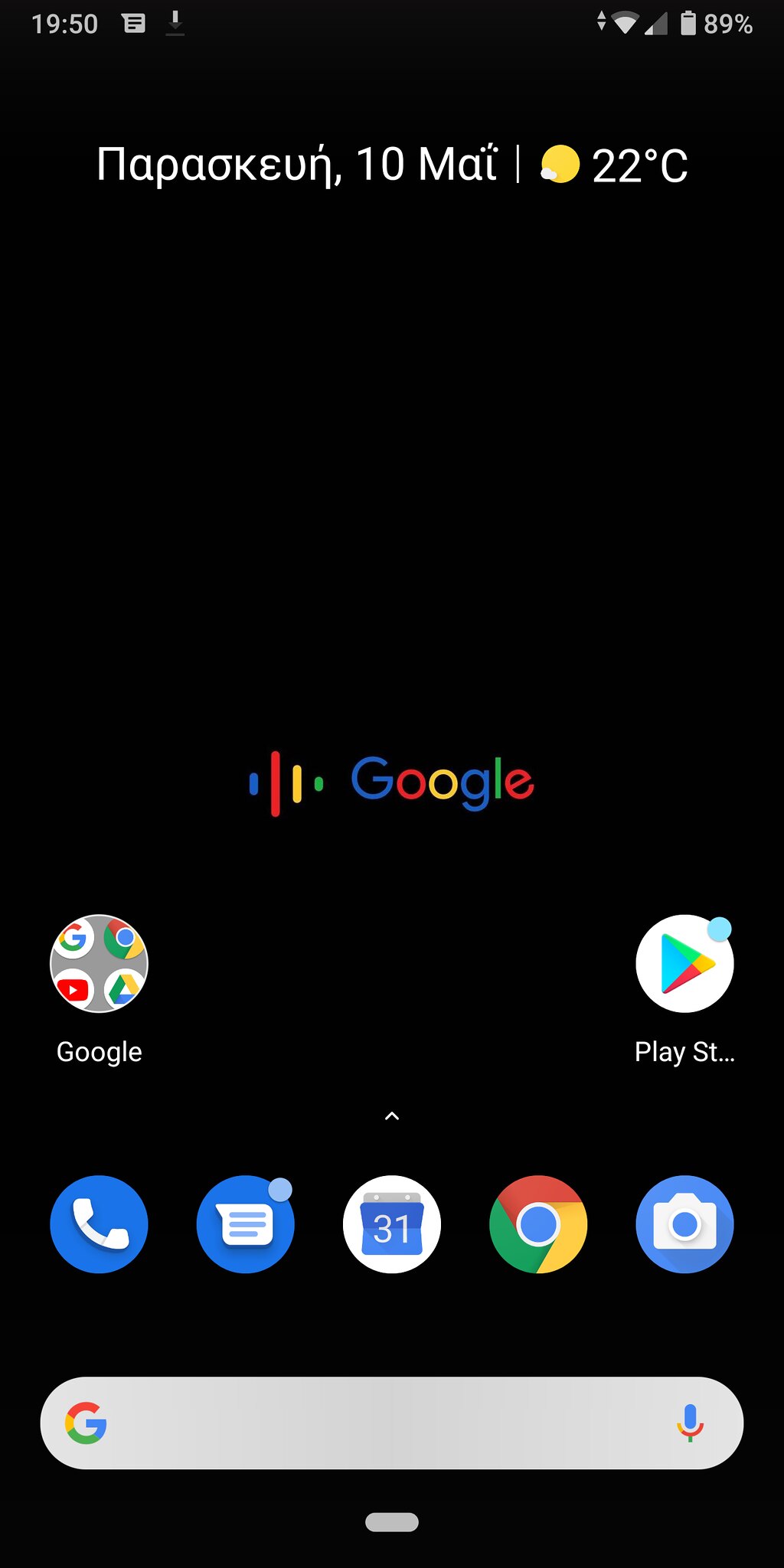This image is a mobile screenshot from an Android phone with a black wallpaper. At the top of the screen, there is a prominent Google logo. Positioned on the far left of the top row is a folder labeled "Google" containing apps like Gmail, Chrome, YouTube, and Drive. On the far right of this row is the Google Play Store icon. 

The second row consists of five neatly arranged icons:
1. A phone icon with a blue background and a white telephone handset.
2. A messaging app icon, which is not descriptively detailed.
3. A calendar app icon.
4. The Chrome browser icon, characterized by its circular shape and tricolored segments of red, yellow, green, with a central blue circle.
5. A camera app icon with a blue background, featuring a white camera symbol and a blue lens.

Beneath these icons, there is a Google search bar. To the left of the search bar is the Google logo, and to the right is a microphone icon, indicating voice search capability.